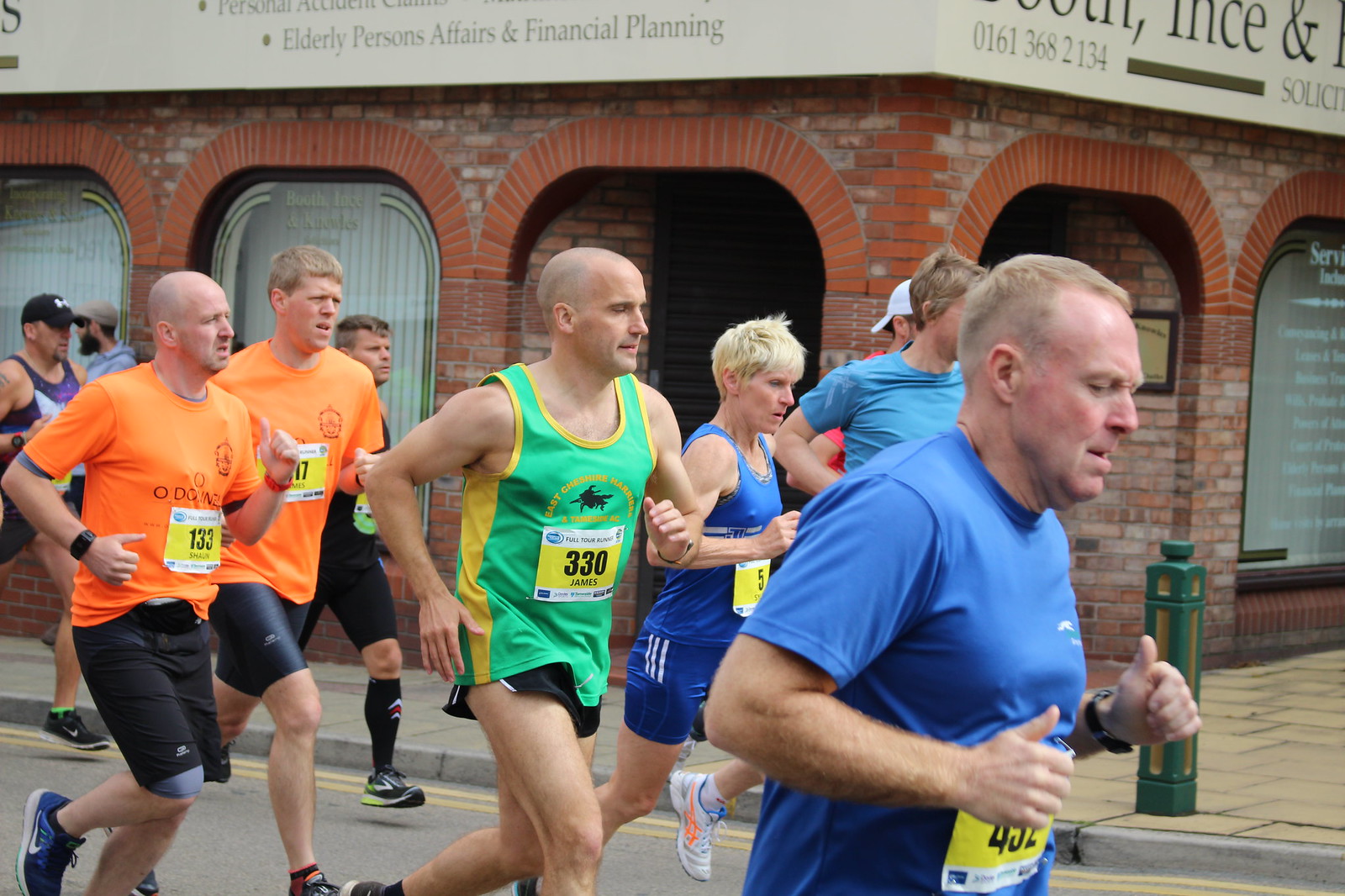The image captures a moment in the midst of a long-distance race on a city street, featuring nine determined runners. In the foreground, an older Caucasian man in his 50s, clean-shaven and dressed in a blue t-shirt with the number 452 on a red tag, leads the group. He is captured in mid-stride with his bent arms indicative of his running motion. Behind him, a young Caucasian man in his 20s or 30s, with a shaved head, wearing a green and yellow tank top and black shorts, follows closely. His tag reads 330. Beside him, a blonde woman with cropped hair, donning a dark blue tank top and navy shorts with white stripes, runs with her number partially obscured. Further back, two men in orange t-shirts and black shorts run in tandem. The foremost of these two, bald and clean-shaven, wears the number 133, while the second, a younger reddish-blonde man, has a matching yellow tag. All runners sport distinct expressions of determination. They stride past a red brick building with a light gray facade, bearing the sign "Elderly Persons Affairs and Financial Planning," partly obscured by the image's framing. The scene is set against the backdrop of urban architecture, with the runners captured from midsection to head, all moving to the right along a brick-tiled sidewalk.